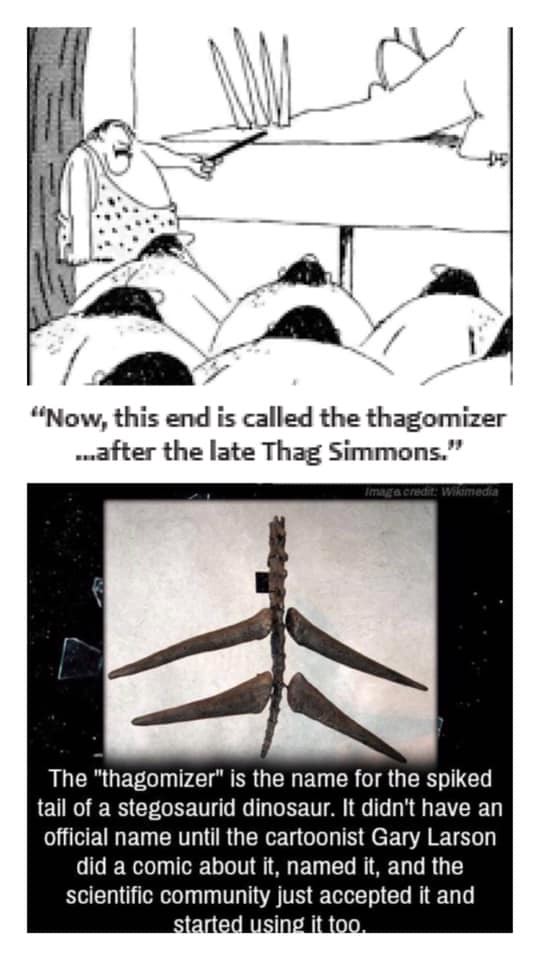The image consists of two sections stacked vertically, each focusing on the tail of an ancient Stegosaurus dinosaur. The upper section is an animated black-and-white cartoon featuring a heavyset man dressed in a caveman costume. He is pointing at what appears to be bones while other cavemen watch in the background. Below this scene is a caption that reads: "Now, this end is called the Thagomizer, after the late Thag Simmons."

The lower section is a plain image with a black background showcasing an object accompanied by text. This text explains that the "Thagomizer" is the name given to the spiked tail of a Stegosaurus. This term was coined by cartoonist Gary Larson in a comic, which the scientific community subsequently adopted as the official name.

In summary, the image illustrates the origin of the term "Thagomizer" for the Stegosaurus' spiked tail, with the upper animated cartoon depicting the moment it was humorously named, and the lower section providing historical context about its acceptance into scientific terminology.